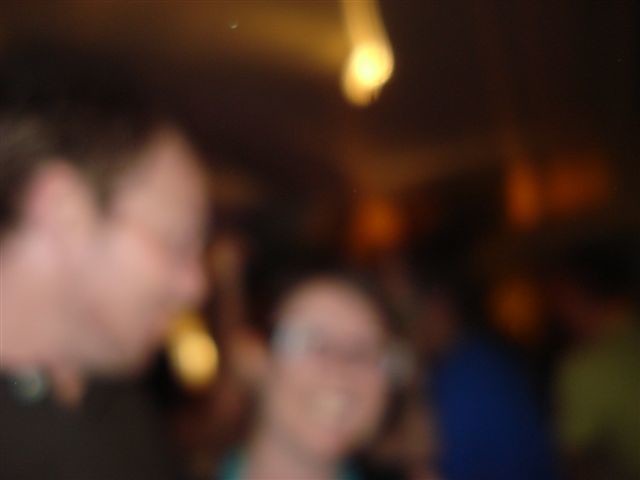The image depicts a somewhat blurry, interior scene with a square composition. At the top of the frame, a dim white light is visible emanating from the ceiling, casting a soft glow over the room. On the left side of the image stands a person, possibly wearing a black sweater and glasses, and sporting short hair. They appear to be gazing to the right.

In the center of the photograph is another person, who is looking directly at the camera with a confident smile. This individual is wearing glasses and a green shirt. To their right, there appears to be a blue object or element in the background.

The background includes an orange-lit wall, partially obscured by a dark ceiling. In addition, there is a black doorway visible in the distant background. Several other people can be seen standing around, though their details are less distinct due to the blur in the image.